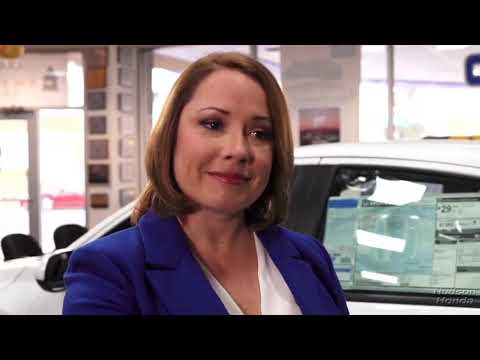This is a detailed photograph of a Caucasian woman taken indoors, likely at a car dealership. The woman, positioned centrally in the image, is captured from her upper chest upwards. She has thin, shoulder-length, side-parted brown hair and is wearing subtle red lipstick. The attire consists of a white v-neck blouse underneath a blue-purple dress jacket. She is smiling slightly and looking over her right shoulder, her body angled towards the right side of the picture. The setting behind her includes a white four-door sedan with visible paperwork in the window indicating vehicle details. Further background elements reveal an indoor structure with a clear glass door on the left and large windows on the right. The photograph itself, which measures about 3 inches wide and 2 inches tall, has narrow black horizontal strips at both the top and bottom, framing the image.